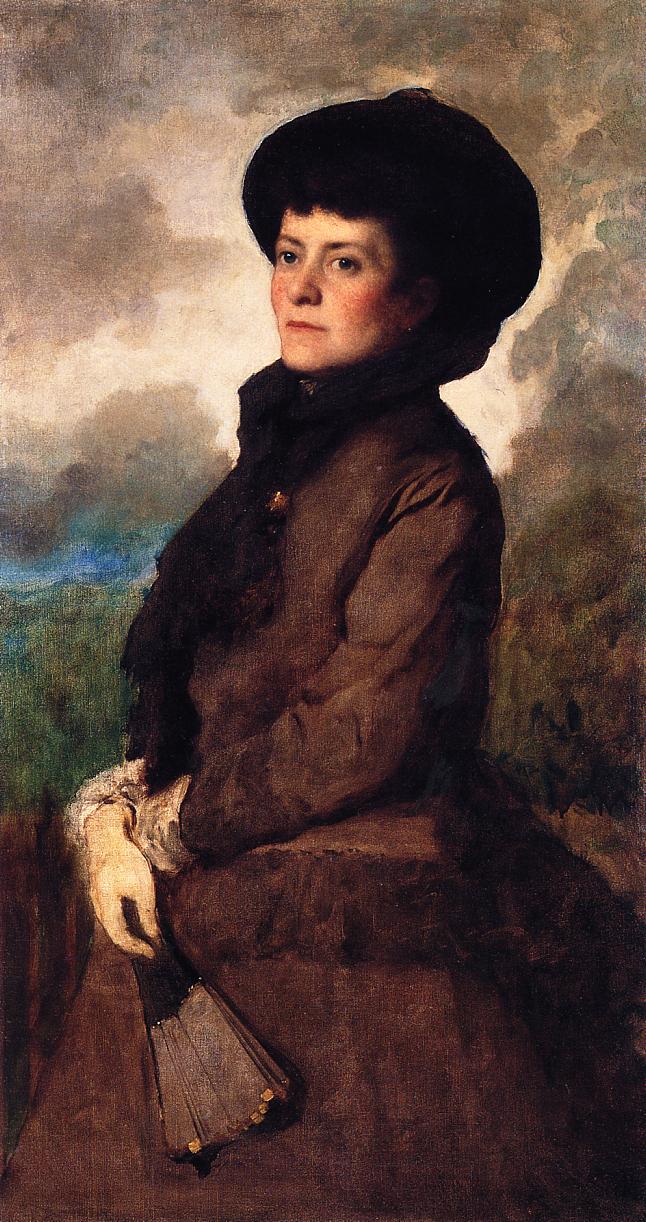This highly detailed painting depicts a Caucasian woman, seen from her mid-thigh up to the top of her head, set against an abstract and blotchy background of green at the base transitioning to blue and gray. The setting suggests an outdoor scene with streaks of green resembling grass, blue indicating a body of water, and gray signifying a cloudy sky. The woman, facing left and slightly tilting her head towards the viewer, reveals three quarters of her face. She wears a dark, nearly black hat that blends with her dark hair, and her dark brown eyes are complemented by rosy cheeks and thin-set lips. She is dressed in an 18th or 19th-century European style, featuring a dark gray dress with a black shawl around her chest. Lace details are visible at her wrists. Her right hand, positioned over her left hand, holds a fan with a black base and gray extensions. The lighting in the painting appears to focus on her face, enhancing her pale skin and straight nose amidst the indistinct, brownish-gray sky backdrop.